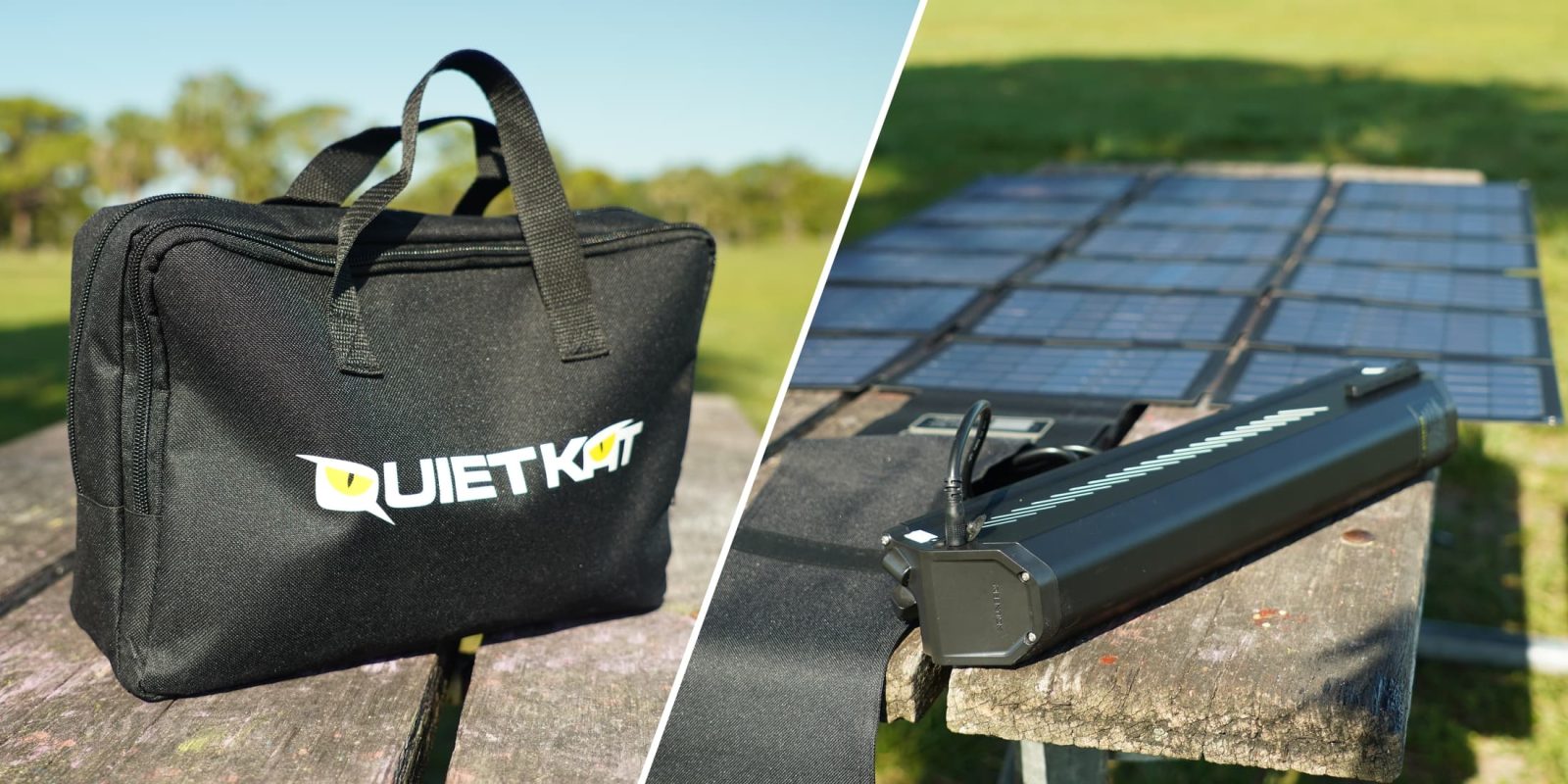This photograph showcases a neatly arranged scene split diagonally into two sections. On the left side, a black bag with black stretchy handles sits prominently on a wooden picnic table. The bag features the white text "QUIET KAT," with the letters Q and A accented in yellow. Behind it, lush green grass and trees stretch into the background under a clear blue sky, creating a serene park setting. On the right side, a sleek, rectangular solar panel is also placed on a similar picnic table. In front of the solar panel, closer to the viewer, there's an additional device that appears to be a power charger. The table surface displays distinct shadows, possibly cast by nearby trees. Overall, the image captures a tranquil outdoor environment with elements suggesting a portable, solar-powered setup, likely aimed at promoting eco-friendly outdoor accessories.